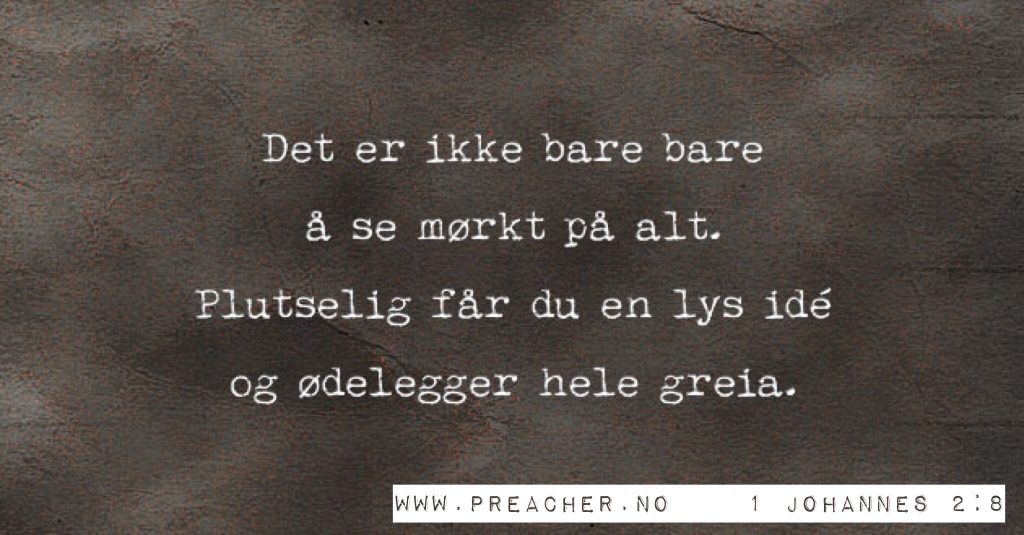The image features a grayish, stone-like background textured with cracks and varying shades of gray, giving it a rugged, almost concrete-like appearance. Overlaying the background is four lines of white text, centered and left-aligned, written in a foreign language, likely Norwegian. Each line of text appears to be a part of two sentences, indicated by periods on the second and fourth lines. In the bottom right corner, there is a white rectangular bar containing dark text that reads "www.preacher.no," followed by "1 Johannes 2:8," suggesting a reference to a biblical verse from 1 John 2:8. The overall layout creates a visual impression of a religious or inspirational message delivered in a structured and formal manner.